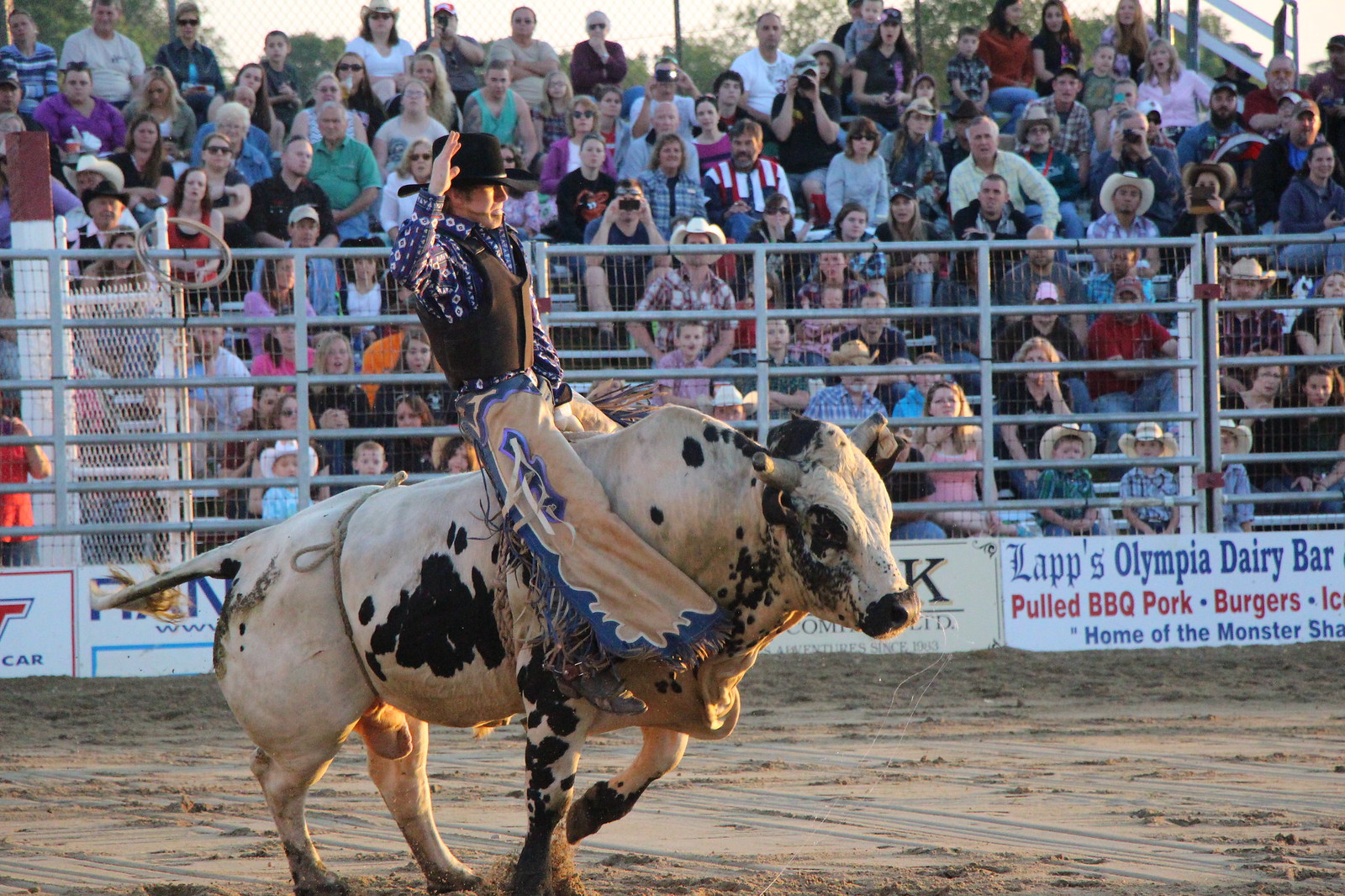In this dynamic photograph, a cowboy is riding a white bull with black spots in a rodeo arena. The cowboy, sporting a black hat, black vest, blue shirt, and cream and blue pants, energetically holds his right arm aloft as the bull leaps mid-stride across the sandy, slightly damp ground. The scene is lit as the sun starts to set, casting warm hues over the arena. Beyond the silver metal fence that marks the boundary of the rodeo ground, a crowd of spectators watch the action intensely. The background features signage from sponsors, including a dairy bar promoting cold barbecue and burgers, catering to a diverse audience enjoying the show.